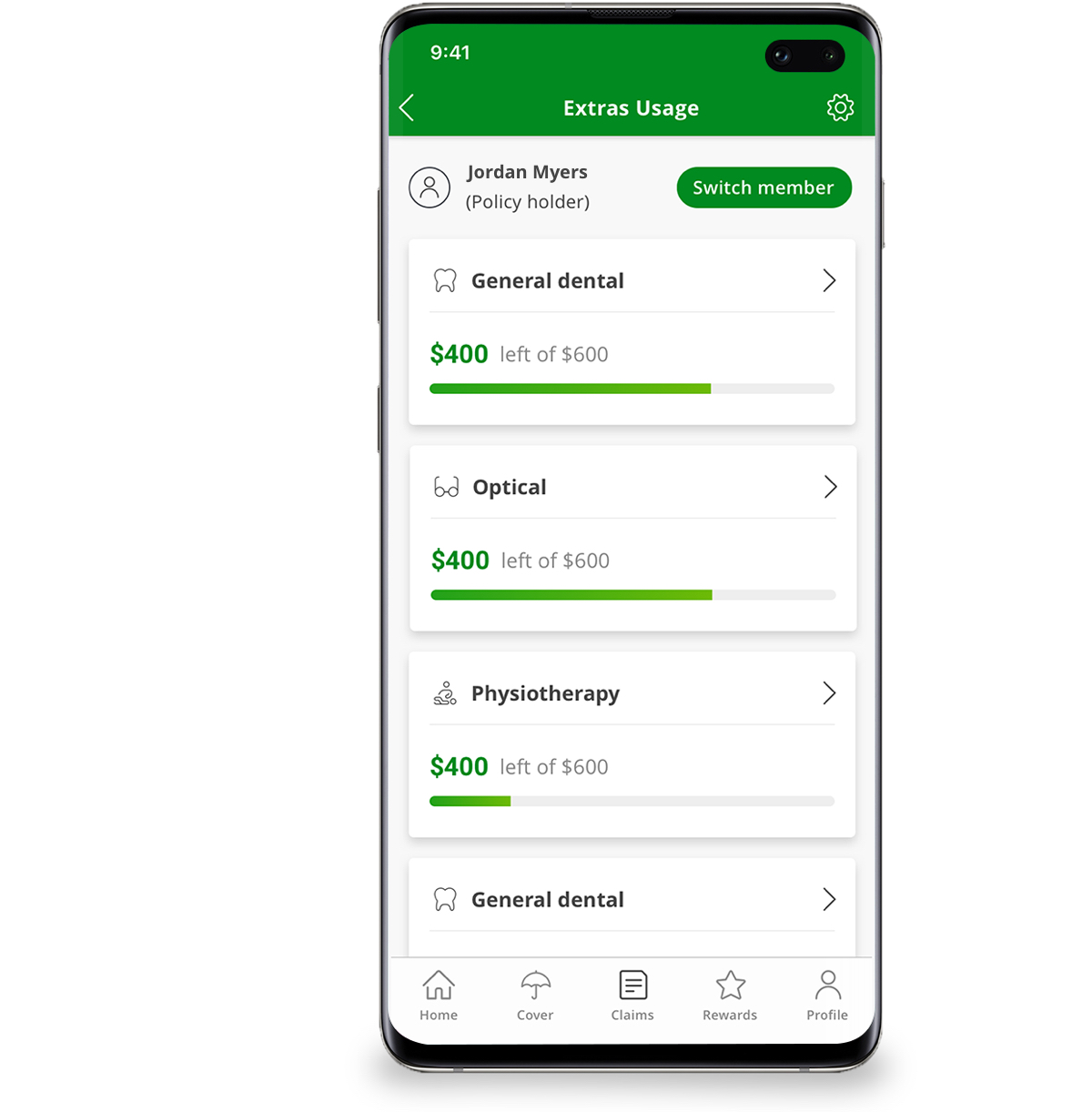The smartphone featured in the image has sleek, silver metallic edges, giving it a high-end appearance. The top section of the screen displays a price of $9.41. Just below, there's a brush with an opal finish featuring a camouflage pattern. There is an arrow indicating a section to select.

Further down, there are additional options labeled "Extras Usage." Towards the bottom of the screen, a gear icon represents a holographic dial. A label on the screen reads “Jordan Meyers (policy holder)” next to a green oval button labeled “Switch Member.”

The interface showcases several rectangular bars with different medical and insurance-related categories:

1. A bar indicating "General Detail Dental" with a value of $400 lifted from a total of $600, represented by a green bar.
2. Another bar labeled "Optical Glasses" with a value of $400 lifted from a total of $600, indicated by a green bar.
3. A third bar labeled "Physiotherapy" showing $400 lifted from $600, again highlighted by a green bar.
4. A fourth bar for "General Dental" also displays a $400 lifted from a $600 limit, showcased by the green bar.

Additional icons near the bottom include:

- A small house icon symbolizing "Home Building."
- An umbrella labeled "Cover."
- A document icon labeled "Claims."
- A holographic dot star labeled "Rewards."
- A person icon indicating "Profile."

Both bottom left and bottom right corners of the screen reflect certain details, suggesting these areas have reflective surfaces.